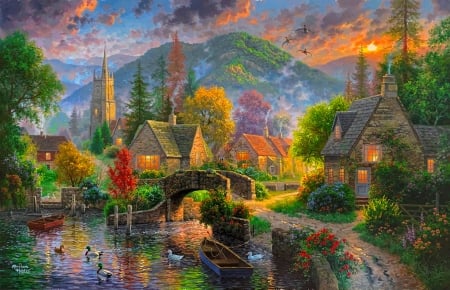This idyllic painting captures a quaint village bathed in the glowing light of either sunrise or sunset, showcasing a blend of soft, warm colors typical of dawn or dusk. Dominating the foreground is a serene pond, home to several lazy ducks and two simple, unoccupied wooden boats, one of which is a notable red. The pond extends into a stream, spanned by a rustic brickwork footbridge. A winding pathway begins at the bottom right and leads towards the bridge, inviting the viewer into the scene. On the left side along the pond, lush vegetation, including vibrant flowers and a variety of trees—some green, others showcasing brilliant reds and yellows—enhances the tranquil atmosphere. 

The middle ground is filled with cozy cottages, their windows glowing with warm light, suggesting the presence of a close-knit community. Among these, a church or cathedral with a tall steeple rises in the background, adding to the rustic charm. Further beyond, the landscape is framed by majestic mountains, their peaks dusted with snow, adding depth to the scene. The sky above is a mesmerizing gradient of blue with golden and orange clouds, reflecting the setting or rising sun that subtly illuminates the peaceful village below.